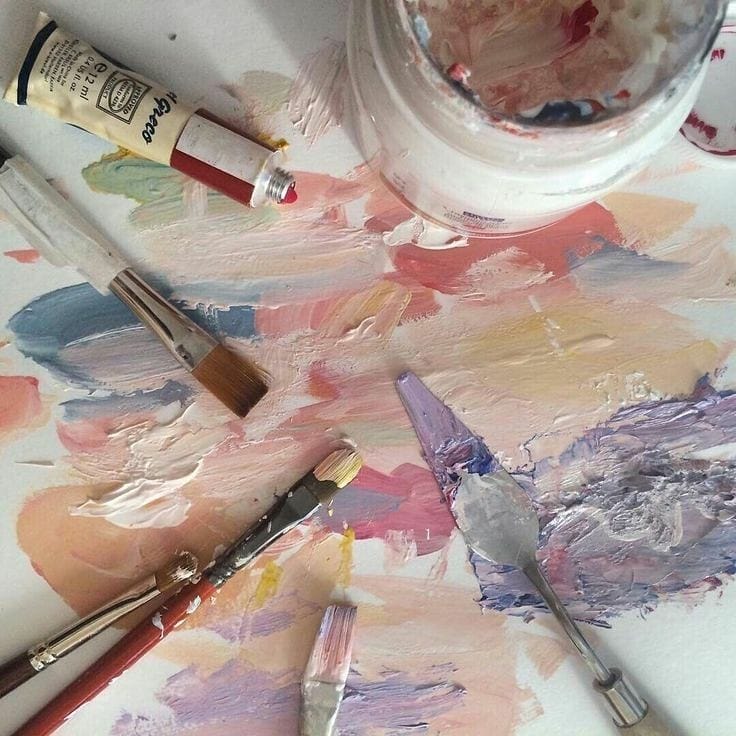This is a detailed, close-up photograph of an artist's workspace as seen from above. Centered on a palette splattered with an array of vibrant colors—purple, peach, pink, blue, and white—the composition captures various paint supplies scattered about. In the upper right corner, a nearly empty glass bottle, once full of white paint, now streaked with multiple colors, hints at ongoing creativity. A tube of red paint with a red and white striped cap and a tan base with black writing, labeled "Greco, 12 milliliters," rests on the palette. Prominently displayed is a thick artist's brush with a metal shaft, laying on its back, while in the lower left corner, two paint-spattered brushes lie with their bristles still coated in paint. Completing the scene, a palette knife smeared with purple paint is positioned in the right center of the image. Altogether, the photograph showcases the dynamic range of materials and paints used, conveying a vivid snapshot of artistic process mid-creation.